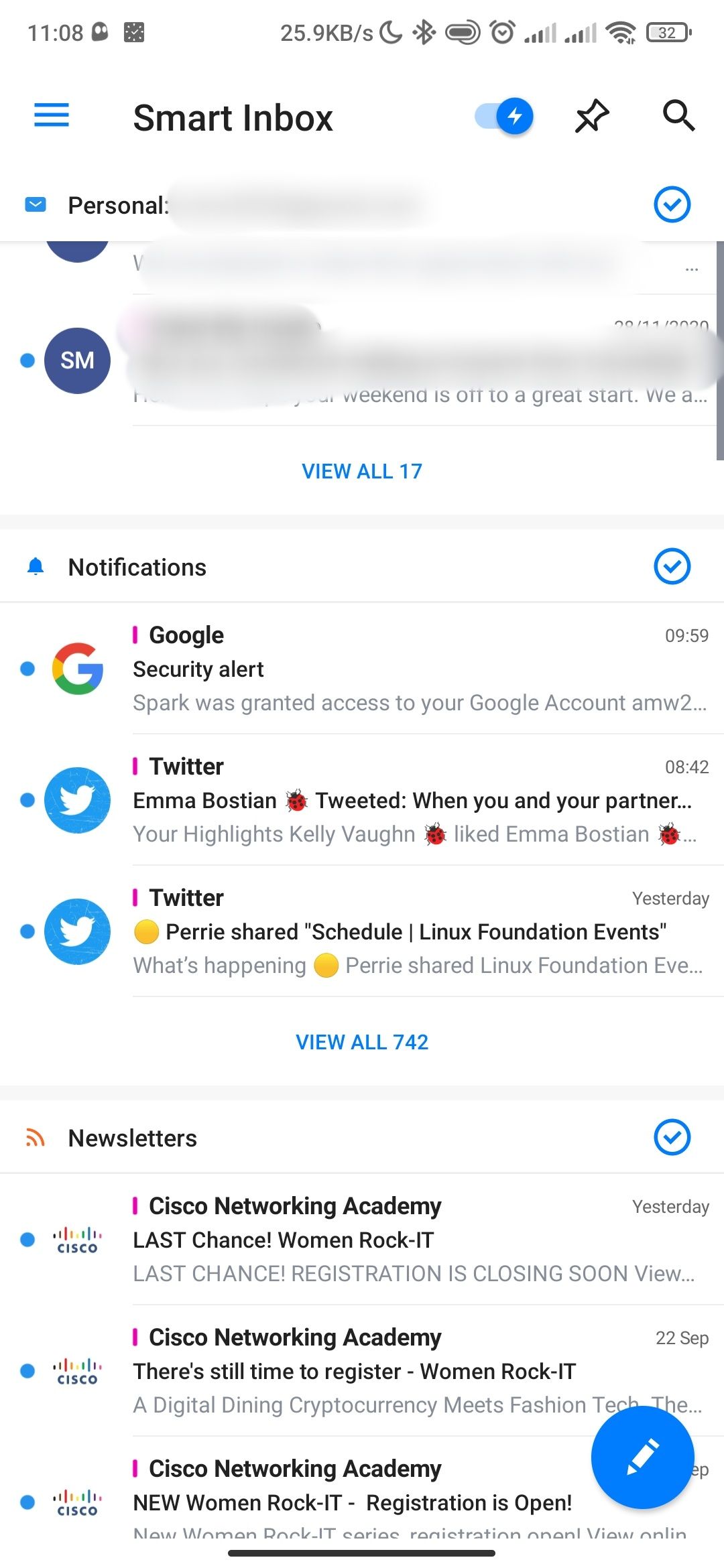The image is a screenshot of someone's smartphone displaying various notifications. At the very top of the screen, the time is shown as 11:08, with a network speed indicator reading 25.9 KB per second. There are several icons present: a crescent moon symbolizing silent mode notifications, an alarm icon, a signal icon, a Wi-Fi icon, and a battery indicator at 32%.

Below this, the title "Smart Inbox" is displayed, indicating the app used to capture the screenshot. Underneath, it says "Personal," with the email address blurred out, followed by blurred content from another email. There's an option titled "View all 17," suggesting more emails are available for viewing.

The next section, marked with a blue bell icon, is labeled "Notifications." The notifications listed include a Google security alert stating, "Spark was granted access to your Google account," followed by truncated text. Further down, a Twitter notification reveals that "Emma Bostonian tweeted," with additional text not fully visible, and another Twitter notification reads, "Perry shared schedule Linux Foundation events."

Below these, there's a prompt to "View all 742" notifications, followed by a section featuring newsletters from Cisco Networking Academy, with three instances visible.